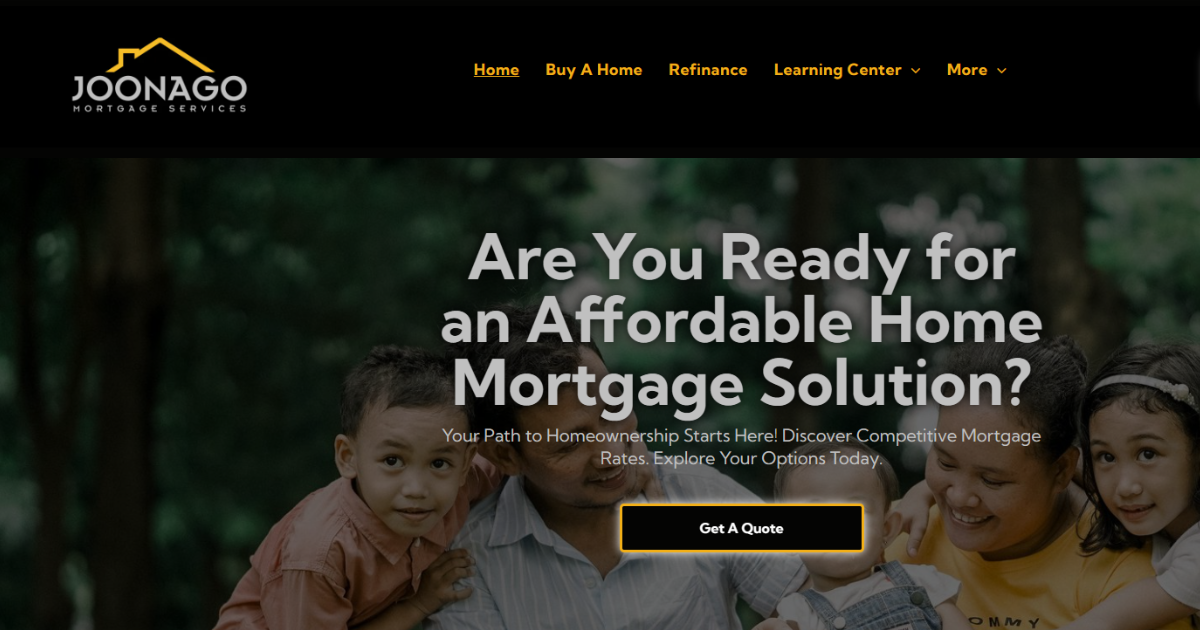The home page of Junago Mortgage Services' website features a prominent black top banner. In the upper left corner, the company's name, "Junago," spelled "J-O-O-N-A-G-O," is displayed in white text, accompanied by an orange outline of a house's ceiling and chimney over the name. Moving to the right-hand side of the banner, there are orange-colored menu options: "Home," "Buy a Home," "Refinance," "Learning Center" with a dropdown arrow for additional choices, and "More," also with a dropdown arrow.

Below the banner, a heartwarming image of a family is showcased, depicting a husband and wife with their three children. From left to right, the son, dressed in a pink collared polo shirt, has his arms on his dad's shoulders and looks directly at the camera. The smiling father, wearing a white striped shirt with rolled-up sleeves, gazes lovingly at his baby daughter in the center, who is clad in a t-shirt and denim overalls. Next to the baby, the mother, wearing an orange t-shirt with black text, shares an affectionate moment while the elder daughter, positioned on the far right, has her arms around her mom's shoulder. This daughter, with long hair and a headband, also looks toward the camera, with the sleeve of her white t-shirt visible. The family is situated in what appears to be a park or forest, evidenced by tree trunks and green foliage in the background.

Superimposed in white text over the image are the words: "Are you ready for an affordable home mortgage solution? Your path to home ownership starts here. Discover competitive mortgage rates, explore your options today." Below this text is a black button with an orange glow around it, featuring the white text "Get a Quote."